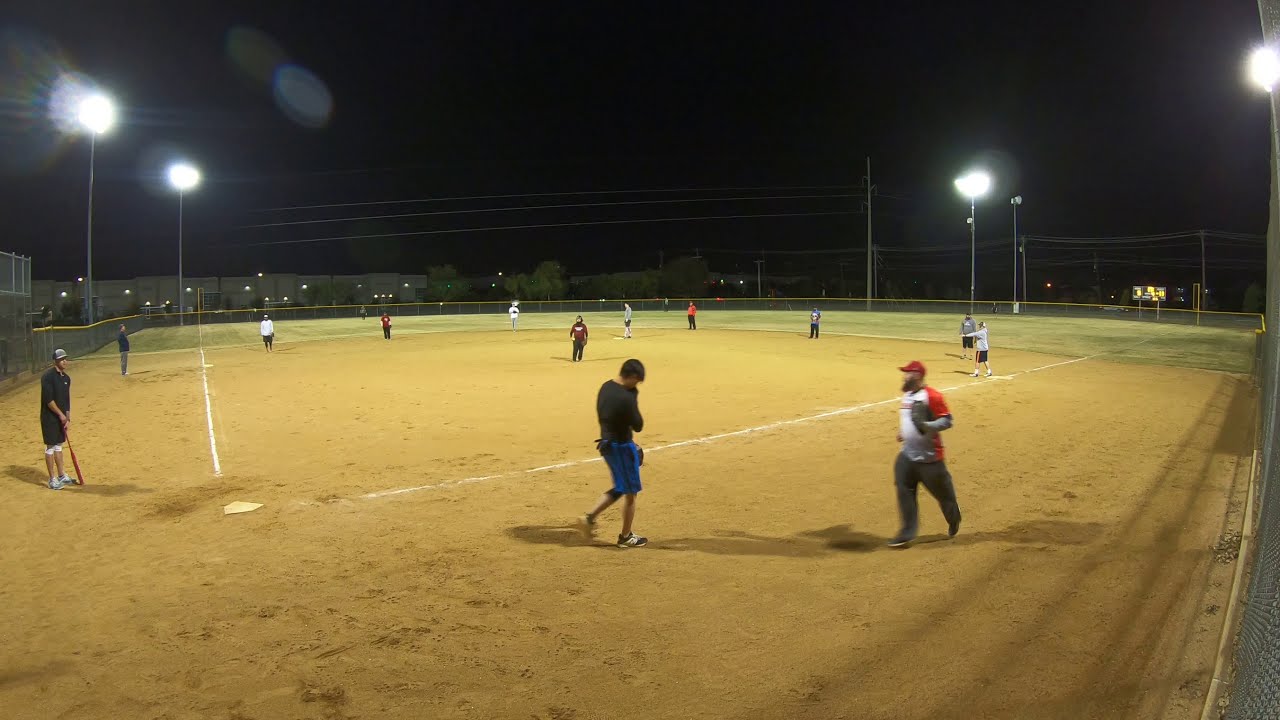The image captures a nighttime baseball game under a starless, dark sky. The upper half of the image is dominated by a connected string of buildings and houses with varying lights, as well as several power line poles silhouetted against the horizon. The lower half reveals a well-lit baseball field with yellow-brown dirt and faint white lines outlining the diamond. 

In the foreground, three players are prominently visible: one in dark pants, a white shirt with red sleeves and back, a red hat, and a beard; another in blue shorts, a dark long-sleeve shirt, and short hair; and a third player on the left wearing a hat, black shorts with white at the bottom, a black shirt, and holding a light tan baseball bat touching the ground. 

Scattered around the field are additional players: one at first base in a white shirt and dark shorts; another in the outfield in a gray shirt and dark shorts; a player near second base in dark pants and an orange shirt; someone between second and third in a gray shirt and dark shorts; another near third base in a colored top, possibly red, and dark pants; and others, including a couple more players in white and dark clothing amidst the positions. 

In the distance, four bright stadium lights—two on the top left and two on the top right—illuminate the scene. While the stands in the background show white dots indicating seats, there are no visible spectators. A fence surrounds the field, particularly prominent on the left side, and a distant scoreboard is visible but unreadable. The overall setting suggests an informal yet engaging nighttime baseball game with no visible umpires.